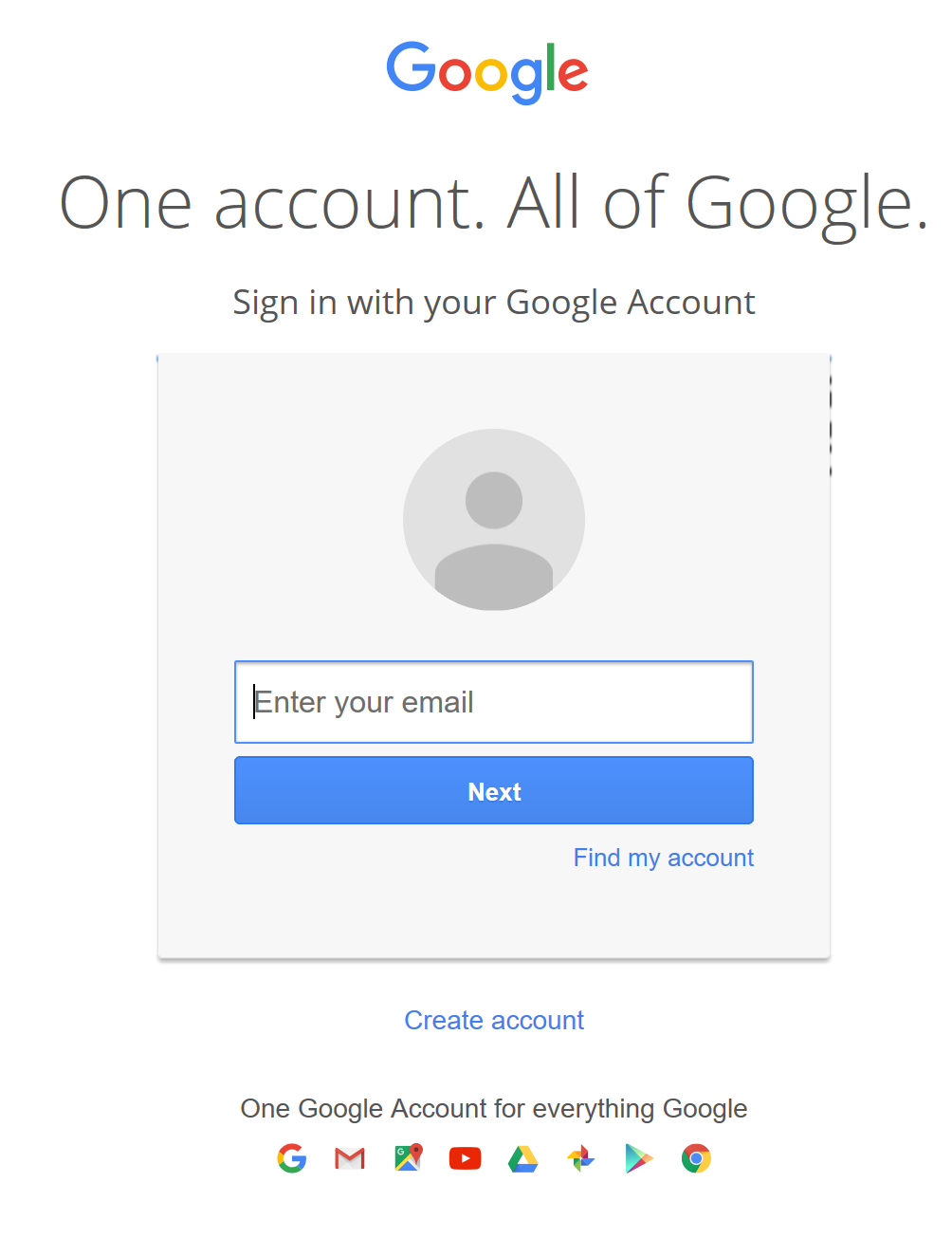The image depicts a Google login page. At the top center of the screen is the bold, colorful Google logo with its iconic blue, red, yellow, and green colors, set against a clean, white background. Below the logo, in the largest font on the page, is the text "One account. All of Google." Beneath this, it says, "Sign in with your Google Account."

Centered below this text is a light gray or off-white square containing a medium and darker gray person icon, which resembles a circle for the head and semi-circular lines for the shoulders. 

Below this icon, there is a white text input box outlined in blue with the placeholder text "Enter your email." Adjacent to this input box is a blue button that says "Next" in white text.

To the right side of the input box, there is a blue "Find my account" link. Just below the input area, there's another blue link that reads "Create account." 

All elements on the page are centrally aligned. Further down, it says, "One Google Account for everything Google," emphasizing the unified nature of Google's services. Below this, a smaller display features icons representing various Google services, including Gmail, Maps, YouTube, Google Drive, Google Photos, the Play Store, and Google Search, each associated with their respective product.